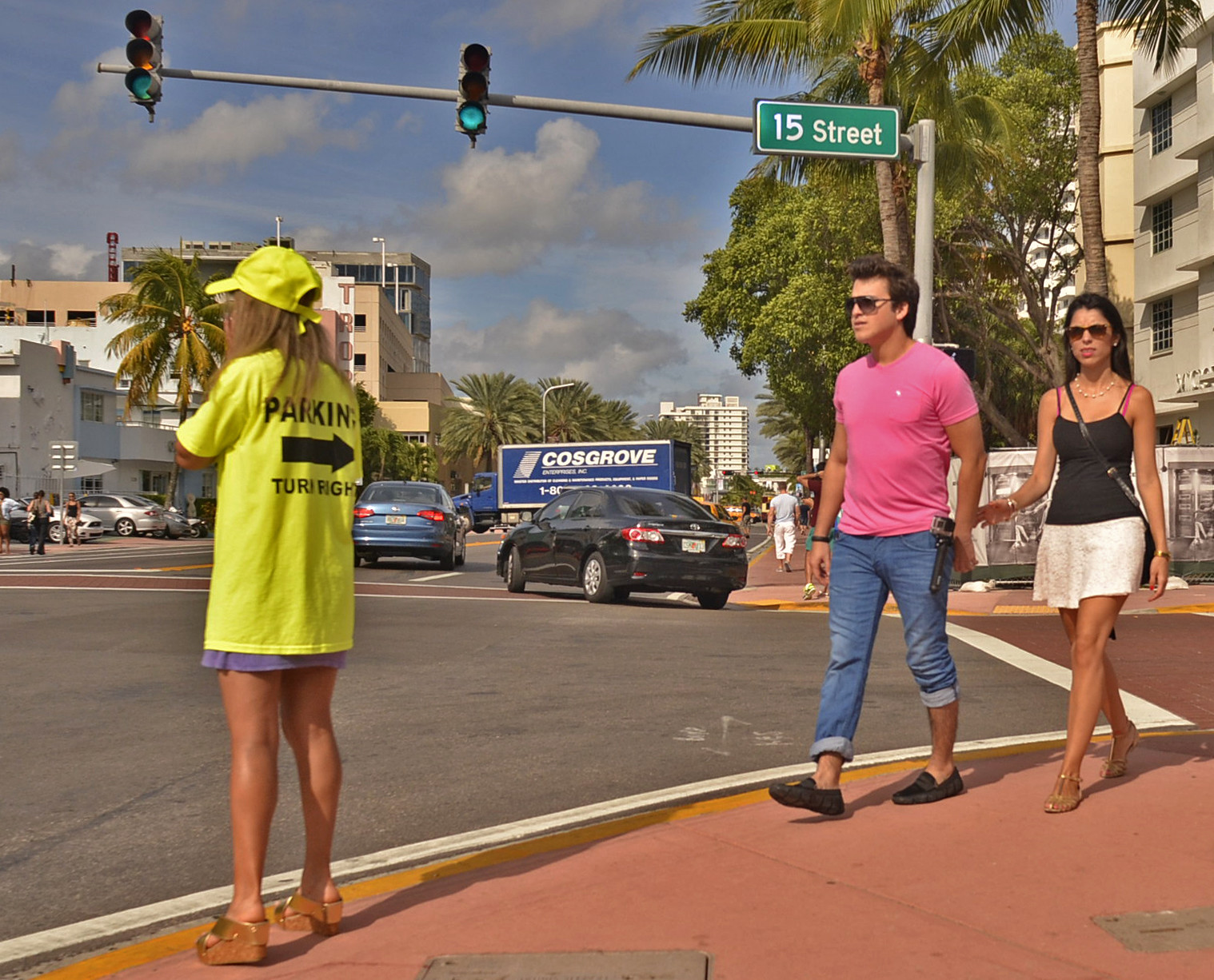In this vibrant city street scene on a sunny day with clear blue skies and fluffy white clouds, three people are walking in the foreground. On the left, a woman faces away, wearing a bright yellow t-shirt and hat, both marked with "parking" and an arrow pointing to the right, indicating directions. She is also in sandals, with her blonde hair partly visible under her hat. On the right, a couple is walking hand in hand toward the woman. The man wears a pink shirt, blue jeans, black shoes, and sunglasses, while the woman beside him sports a black tank top, white skirt, sandals, and a purse slung across her chest. 

The street they walk on is paved with red bricks, bordered by white and beige buildings, palm trees, and other trees in the background, contributing to the scenic beauty. Cars, including a notable blue vehicle and a semi-truck labeled "Cosgrove," navigate the large intersection ahead. A green street sign with "15th Street" hangs from a post above the traffic lights, where the signal is green. The scene is bustling with activity, with additional parked cars, distant pedestrians, and various buildings lining the street, enhancing the urban atmosphere.